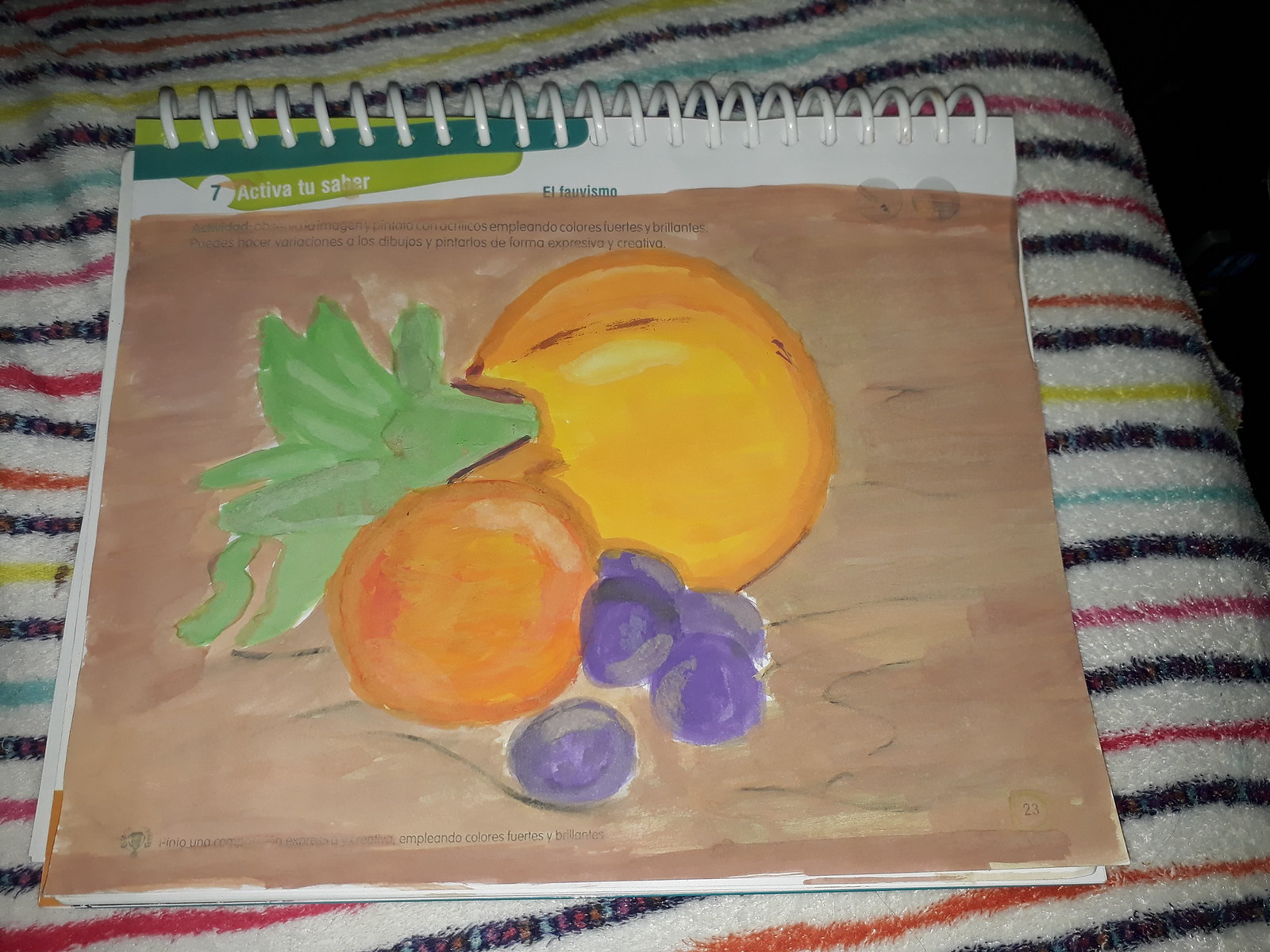This photograph captures a still life painting within an open sketchbook, bound with spiral rings. The sketchbook is placed against a backdrop featuring subtle, horizontal stripes, suggesting a textile such as a towel or blanket. The painting itself is minimalist, set against a tannish-brown background. It showcases a collection of fruit, including a large orange, a tangerine, and five plums, accompanied by a simple green element. The overall style of the painting is basic and lacks intricate details, emphasizing a straightforward, uncomplicated representation.